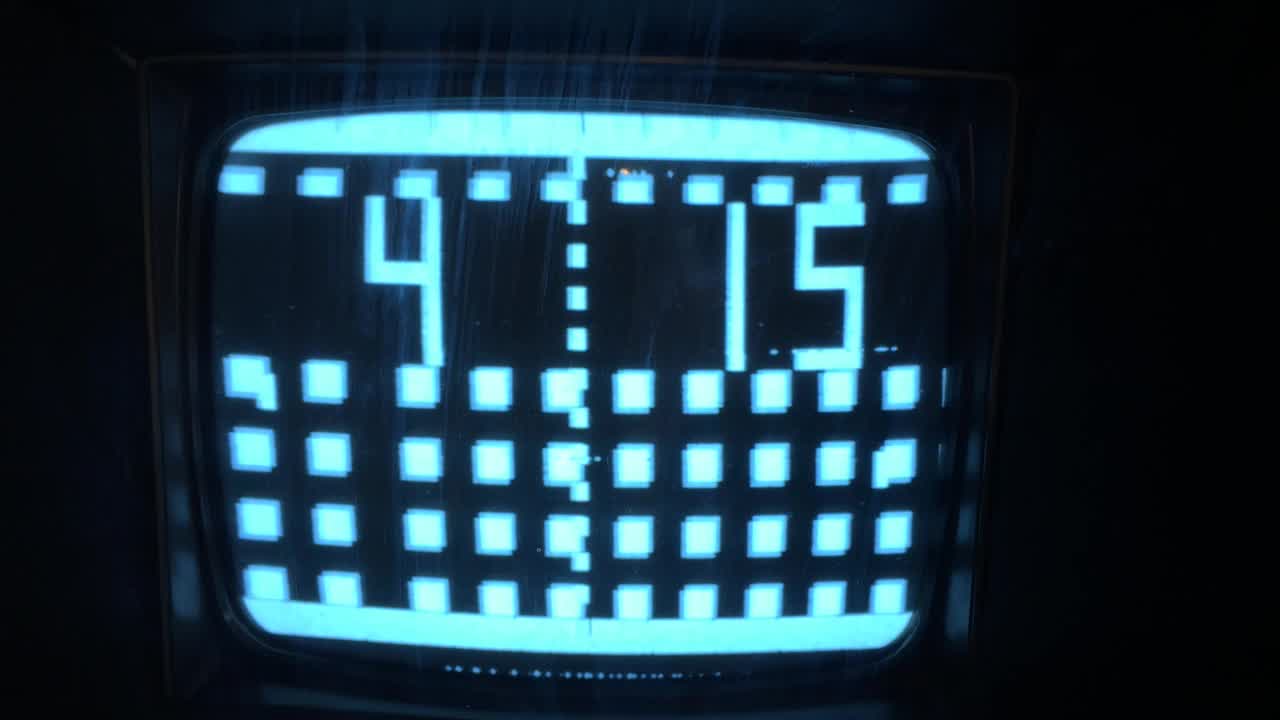A detailed close-up photo of a digital clock, primarily focusing on its screen. The clock is housed in a silver or white plastic frame, though the edges are obscured by deep shadows, making it difficult to discern any further details about its casing. The screen itself glows with a bluish hue, clearly displaying the time "4:15." The display is divided by several prominent blue squares arranged vertically between the hour and the minutes. Along the top edge of the screen, a series of smaller white-blue squares are visible, creating a border effect. Similarly, at the bottom, a sequence of solid blue squares lines the edge. Beneath these, there are ten rows of smaller squares, each consisting of four individual blue squares, adding to the intricate design of the clock's interface.